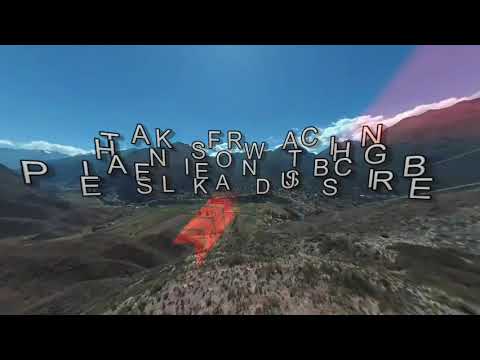The image depicts a mountainous landscape with a valley below, likely seen from an aerial or high vantage point. The valley is rich with greenery, featuring a blend of trees and green fields. The scene is framed at the top and bottom by black stripes, giving it a cinematic feel, akin to the opening of a movie. The serene blue sky is punctuated by clouds hovering above the mountains. On the right side of the image, a ray of reddish light slants towards the bottom, adding a dynamic element.

Dominating the upper middle portion of the picture is a dense array of scrambled letters, seemingly forming a cryptic message or word puzzle that possibly reads "thanks for watching" once deciphered. These letters are scattered and overlapping, creating a challenging visual riddle. Below this, there's a faint holographic image of an orange train and its car, adding to the enigmatic nature of the scene. The spacious, brown-hued terrain is marked by a series of red arrows, either as part of the landscape or superimposed for visual effect, contributing to the picture's intricate and mysterious atmosphere.